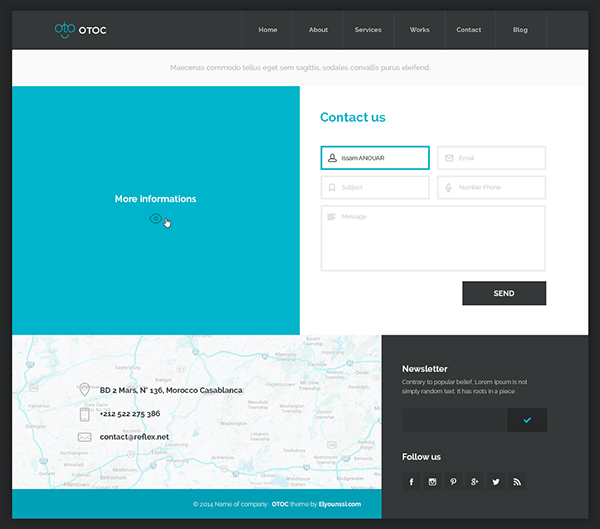The image appears to be a structured layout, possibly a webpage design, with a series of colored sections each containing specific elements. Here's a detailed caption:

---

The image displays a meticulously organized webpage layout with a series of colored sections. At the very top, there is a black square featuring the letters "OTOC" in white, followed by navigation links "Home," "About," "Services," "Contact," and "Blog" in white text, aligned horizontally. Below this, there's a white rectangle containing text in a foreign language.

Directly beneath the white rectangle is a blue and white section divided horizontally. On the left, there is a blue rectangle with the text "More Information" and an eyeball icon, accompanied by a clickable hand icon indicating interactivity. On the right, the white rectangle has "Contact Us" written in blue letters.

Further down, the layout includes another blue rectangle featuring the icon of a person and some content in black text, presumably a person's name although it's not clearly visible. Adjacent to this, there are a series of grey rectangles labeled "Email," "Subject," and "Number/Phone" likely representing input fields. Below these fields, there is a black button labeled "Send."

Towards the bottom, there is a combination of a white and blue rectangle showing a map, and a black square indicating "Newsletter" followed by a small, unreadable paragraph. Lastly, the text "Follow Us" suggests links to social media or additional contact options.